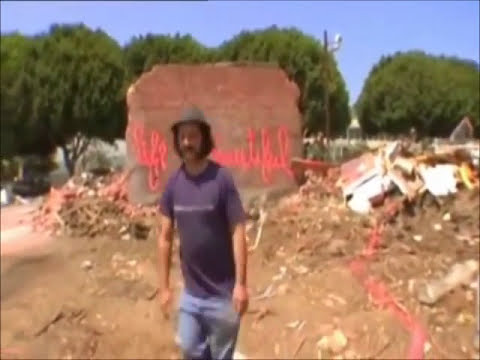In this sunny, outdoor setting captured in a low-resolution photograph, a Caucasian man stands amidst the ruins of a collapsed building, its rubble scattered across the ground. He is dressed in a dark blue or purple T-shirt, blue jeans, and a hat with a rounded brim. The man, characterized by black hair, a black mustache, and possibly long sideburns, is seen in a peculiar posture with arms slightly extended forward. Behind him, amidst the dirt and debris, one wall remains partially standing with red or orange spray-painted graffiti on it. The background reveals a clear blue sky, some tall green bushes, and rounded trees. A telephone pole is also visible in the distance. The image, slightly blurry and soft in detail, appears like a screenshot from a video, contributing to its unfocused and indistinct nature.